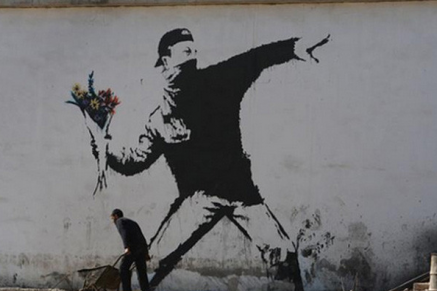This image features a renowned piece of street art by the elusive artist Banksy. It depicts a young man, standing against a white concrete wall, with a scarf covering his lower face and a backwards baseball cap on his head. The man is in a dynamic pose, poised to throw a bouquet of flowers, which he holds in his right hand. The bouquet, comprised of vibrant yellow and red wildflowers, stands in stark contrast to the monochromatic tones of the man and his attire; he is dressed in jeans and a long-sleeve jacket. In front of this evocative mural, a real man is captured pushing a wheelbarrow, adding an element of reality to the striking piece that juxtaposes aggression with symbols of peace and love.